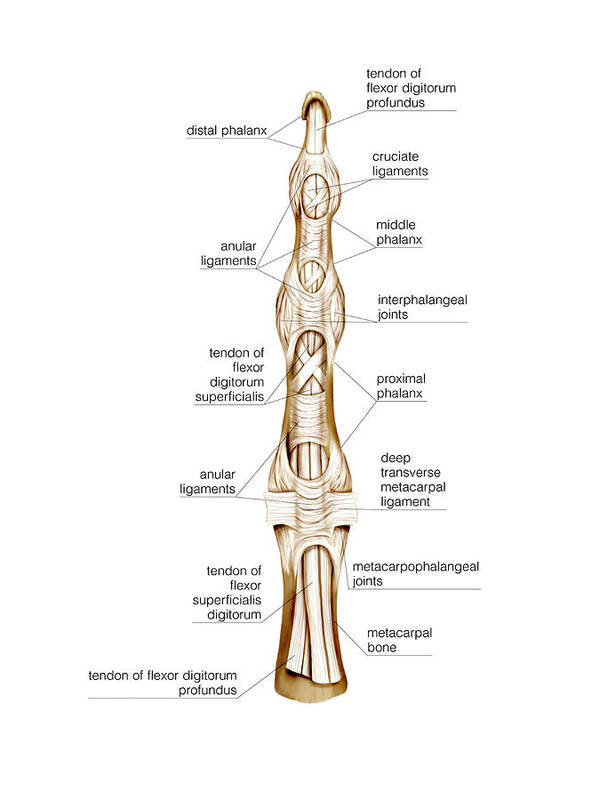The image is a detailed anatomical diagram of the various parts of the finger muscles and tendons. At the top, it illustrates the "Tendon of Flexor Digitorum Profundus" followed by the "Distal Phalanx," "Cruciate Ligaments," and "Middle Phalanx." Further down, it marks the "Interphalangeal Joints" and the "Tendon of Flexor Digitorum Superficialis." The "Proximal Phalanx" and "Annular Ligaments" are also highlighted, followed by the "Deep Transverse Metacarpal Ligaments." The diagram continues with the "Metacarpophalangeal Joints," the "Tendon of Flexor Superficialis Digitorum," and the "Metacarpal Bone." Finally, the "Tendon of Flexor Digitorum Profundus" is labeled again at the bottom. The bones and tendons appear primarily white with some brown hues, indicating their respective textures and structures. This comprehensive illustration is characteristic of an A&P Anatomy and Physiology textbook.